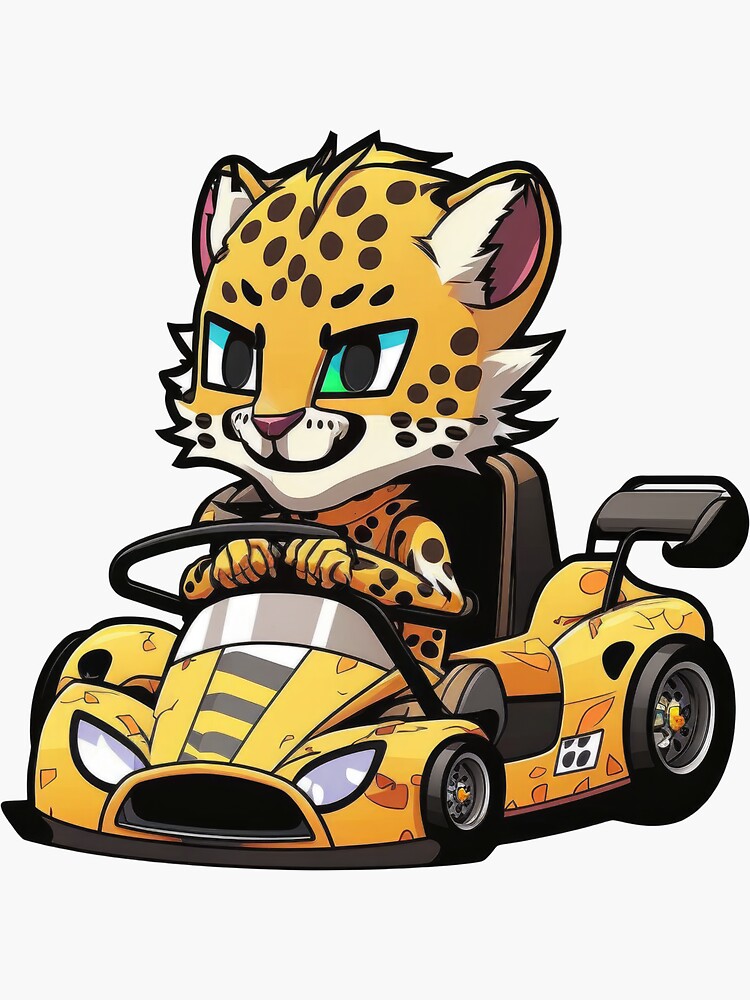A vibrant, whimsical illustration features a cartoony cheetah seated inside a race car, adding a playful twist to the animal's signature speed. The cheetah, predominantly orange with contrasting white around its muzzle and mouth, is depicted with narrowed eyes and a cheerful smile, radiating confidence and excitement. Its fluffy ears stand out as it firmly grips the steering wheel, prepared for a thrilling drive. The race car, painted in a matching orange hue with bold black stripes adorning the hood, exudes a sleek and speedy aesthetic. Enhanced with a black spoiler and larger back tire for high performance, the car sits prominently against a spotless white background, devoid of any text, people, or environmental elements. The simplicity of the backdrop focuses attention solely on the dynamic and lively character, capturing a moment of spirited adventure in a minimalist setting.